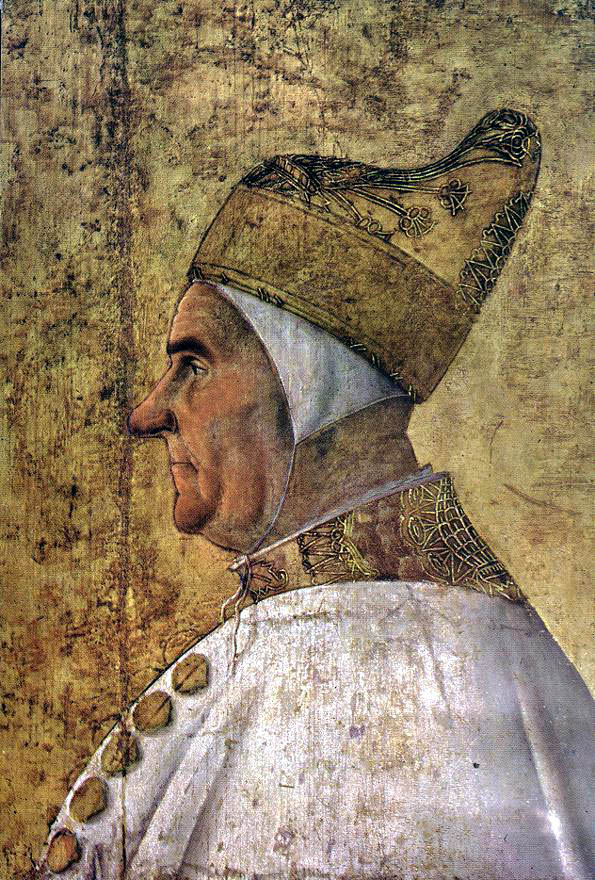This intricate artwork, likely from the Renaissance or earlier, depicts an elderly clergyman in a detailed side profile. He is adorned in a white robe featuring large, ornate gold buttons from the neck down his chest. Around his neck and at the collar, there are lavish gold embellishments. His head is covered by an interestingly shaped, ornate gold headpiece that curves and sticks up in the back, resembling a modern boot in design. Beneath this headpiece, a white cloth with a strap is visible, encircling his neck. The clergyman's facial features are distinct and expressive, with pronounced wrinkles on his forehead, bushy eyebrows, a pronounced pointy nose, and a notably hefty, full neck. The backdrop is a distressed, gold-toned surface interspersed with dark flecks and shadows, adding depth and texture to the image's overall composition.